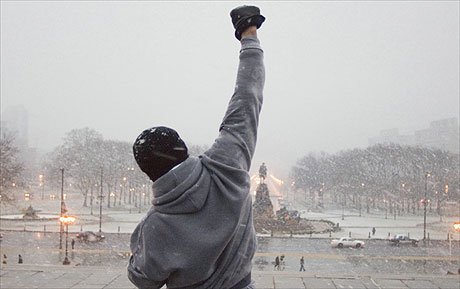In this iconic scene from the movie "Rocky," the famous character stands triumphantly at the top of the steps of the Philadelphia Museum of Art, viewed from behind. Rocky, dressed in a gray hooded sweatshirt and sporting a black beanie and black gloves, raises his right arm victoriously into the air. The camera captures him from the waist up, looking out over the cityscape that is blanketed in heavy snow. 

Below, cars drive along the snowy roads, and a monument stands prominently amidst a wintry scene filled with people walking by. The sky is an overcast gray, casting a monochromatic tone over the city. Trees in the distance are dark but outlined with snow, contributing to the cold and bleak atmosphere. Streetlights cast a faint yellow glow despite the heavy snowfall, and the wet pavement, marked by a distinctive yellow line, reflects the scene’s cold, somber mood. This moment encapsulates Rocky's perseverance and determination, set against the backdrop of a dreary and challenging winter day.